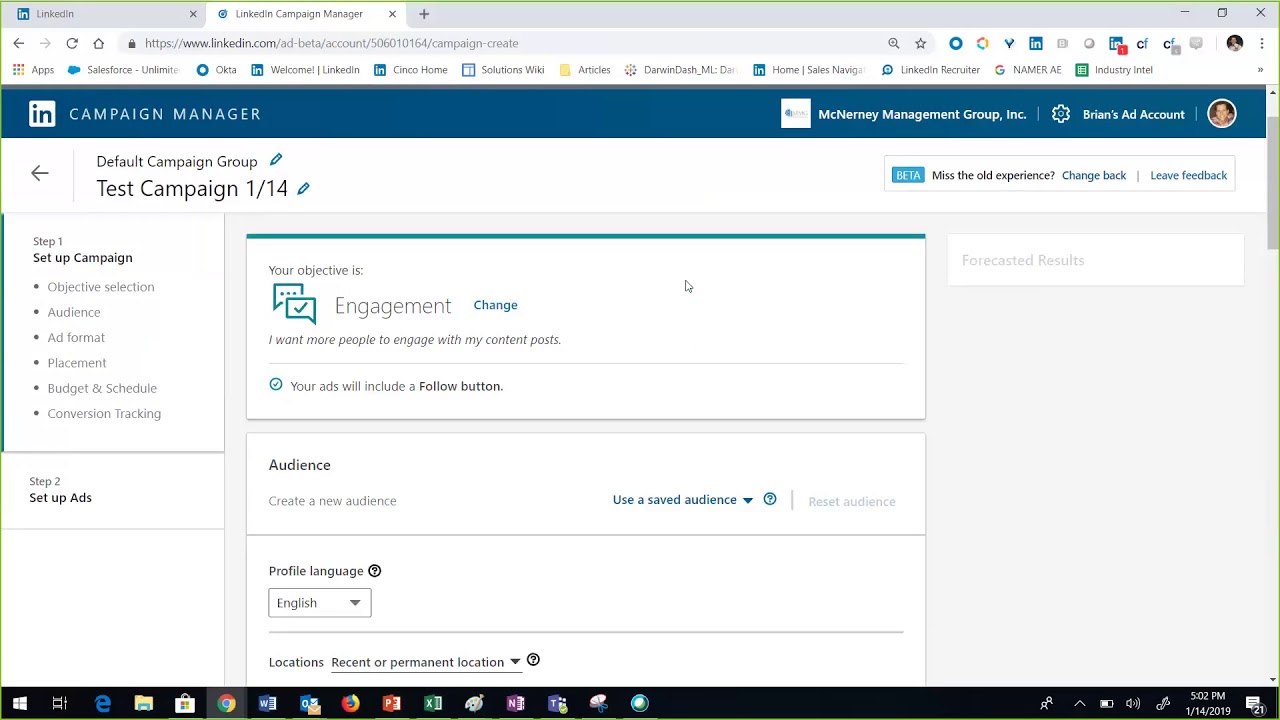This screenshot captures the interface of LinkedIn's Campaign Manager. At the top, there are two taskbars visible: one for LinkedIn and another for LinkedIn Campaign Manager. The search bar displays the URL: `https://www.linkedin.com/ad-beta/account/506010164/campaign-create`.

In the blue bar at the top of the screen, it specifies the application as "Campaign Manager" and next to this is the account name "McNearney Management Group Inc." To the right, it indicates "Brian's ad account" accompanied by a settings gear icon.

The interface detail shows a hierarchical structure starting with "Default Campaign Group" followed by "Test Campaign 114." Below this, the screenshot shows a progression bar labeled "Step 1: Set Up Campaign," which includes stages like "Objective Selection," "Audience," "Ad Format," "Placement," "Budget and Schedule," and "Conversion Tracking." The subsequent step, "Step 2: Set Up Ads," is also displayed.

To the right, it indicates that the current campaign objective is "Engagement," which the user can change. The note specifies, "I want more people to engage in my content tasks," and mentions that the ad will include a follow button.

Further details include options for "Audience," where users can create a new audience or use a saved one. Users can also specify "Profile Language" and select "Location," with options for "Recent or Permanent Location" from a drop-down menu.